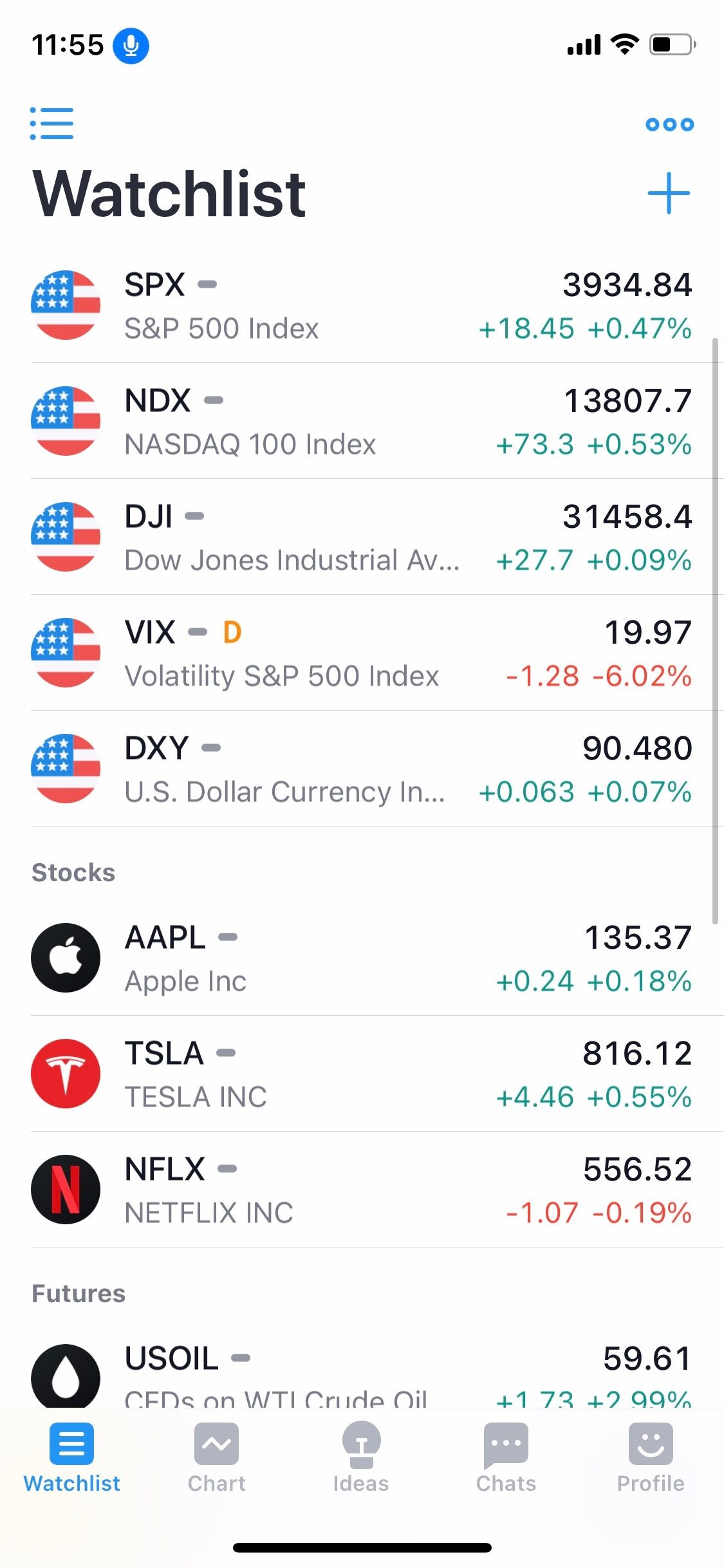This is a screenshot of a stock exchange application interface. In the top left corner, there is a section labeled "Watchlist" in black text. Listed vertically beneath this heading are various company stocks, with most stock prices trending upward, aside from two that are declining.

Below the Watchlist, there is another section labeled "Stocks." Although this heading is not in black text, it clearly includes the abbreviated ticker symbols for companies like Apple (AAPL), Tesla (TSLA), and Netflix (NFLX).

The interface also displays several key stock indices and prices: 
- S&P 500 (SPX) at $3,934
- NASDAQ 100 (NDX) at $13,807
- Dow Jones Industrial Average (DJI) at $31,458
- Volatility Index (VIX) at $19
- US Dollar Index (DXY) at $90

Additionally, it shows the current stock prices for individual companies:
- Apple (AAPL) at $135
- Tesla (TSLA) at $816
- Netflix (NFLX) at $556